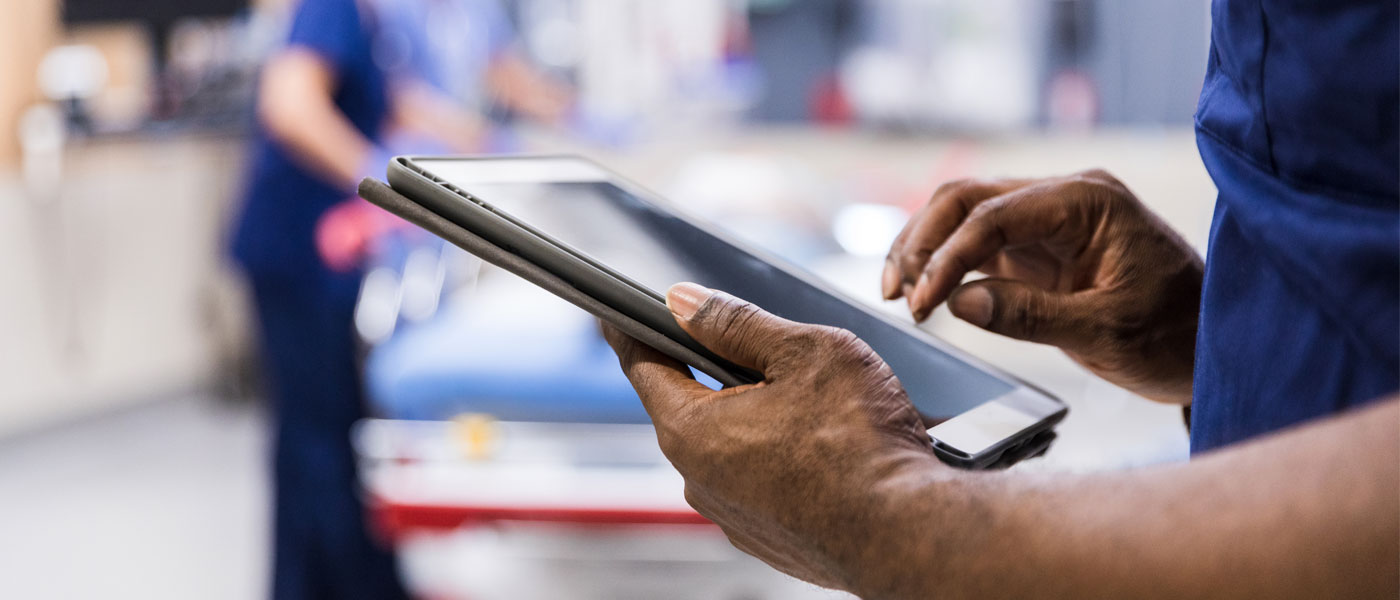In this vivid and detailed image, an African-American man, clad in navy blue scrubs, holds a rectangular tablet in his left hand while his right hand hovers over the screen, ready to touch it. The man’s dark blue attire contrasts sharply with the blurry background, accentuating his presence and the device. In the backdrop, hinting at a hospital setting, another person, also in navy blue scrubs, stands with her bare arms visible, suggesting she might be a medical staff member. The background features a hospital bed without a patient, sporting a modern design with a red trim and a light blue mattress, and possibly a desk or medical counters on the side. Additionally, a red object is noticeable amidst the hazy backdrop, further suggesting the clinical environment.